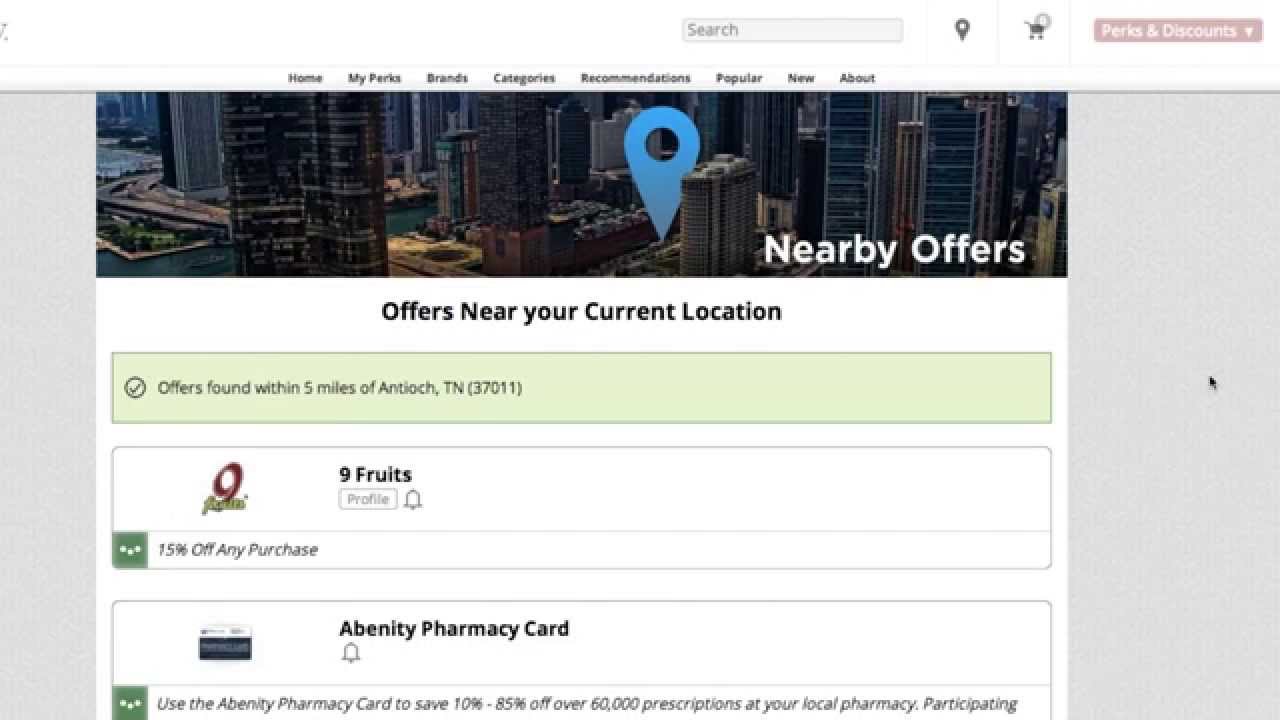This is an image showcasing the user interface of an app named Pitcher. At the very top, there's a prominently placed search bar for users to quickly find specific items. To its right is a shopping cart icon, indicating where users can view their selected purchases. Further to the right, there's a button dedicated to perks and discounts.

Directly below these elements lies a center-justified menu bar with several options: Home, My Perks, Brands, Categories, Recommendations, Popular, and New. Beneath this menu bar is a large banner featuring an aerial view of a city skyline. The perspective is from above, offering a diagonal glance at the tops of buildings, although the tops and bottoms are cut off, providing a dynamic visual of the urban landscape. A blue marker is centrally located within this city snapshot.

Towards the bottom right of the banner, the text "Nearby Offers" is displayed, leading into a white section below that spells out "Offers near your current location." At the very bottom, distinguished by a green bar, the text reads "Offers found within five miles of Antioch, Tennessee 37011," specifying the geographical range of the available offers.